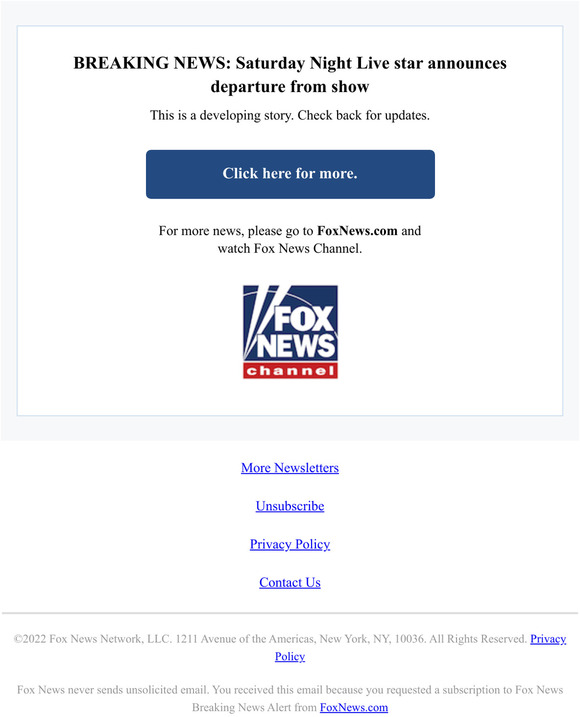This image is a screenshot set against a white background, depicting a section of a website featuring breaking news. At the top of the white box, bold black text reads, "Breaking News: Saturday Night Live Star Announces Departure from Show." Beneath this headline, smaller black text indicates, "This is a developing story, check back for updates." Just below this text lies a prominent blue action button labeled "Click Here for More."

For further updates and information, viewers are directed to "foxnews.com" and encouraged to watch the Fox News Channel. The Fox News Channel logo is situated towards the bottom of the image. The logo comprises a dark blue square with a red banner at the bottom; within the square, "Fox News" is displayed in bold white block text, and the word "Channel" is set against the red banner. The logo also features two beams of light extending from the lower left corner towards the center top.

Below the Fox News Channel logo, there are several links for "More Newsletters," "Unsubscribe," "Privacy Policy," and "Contact Us."